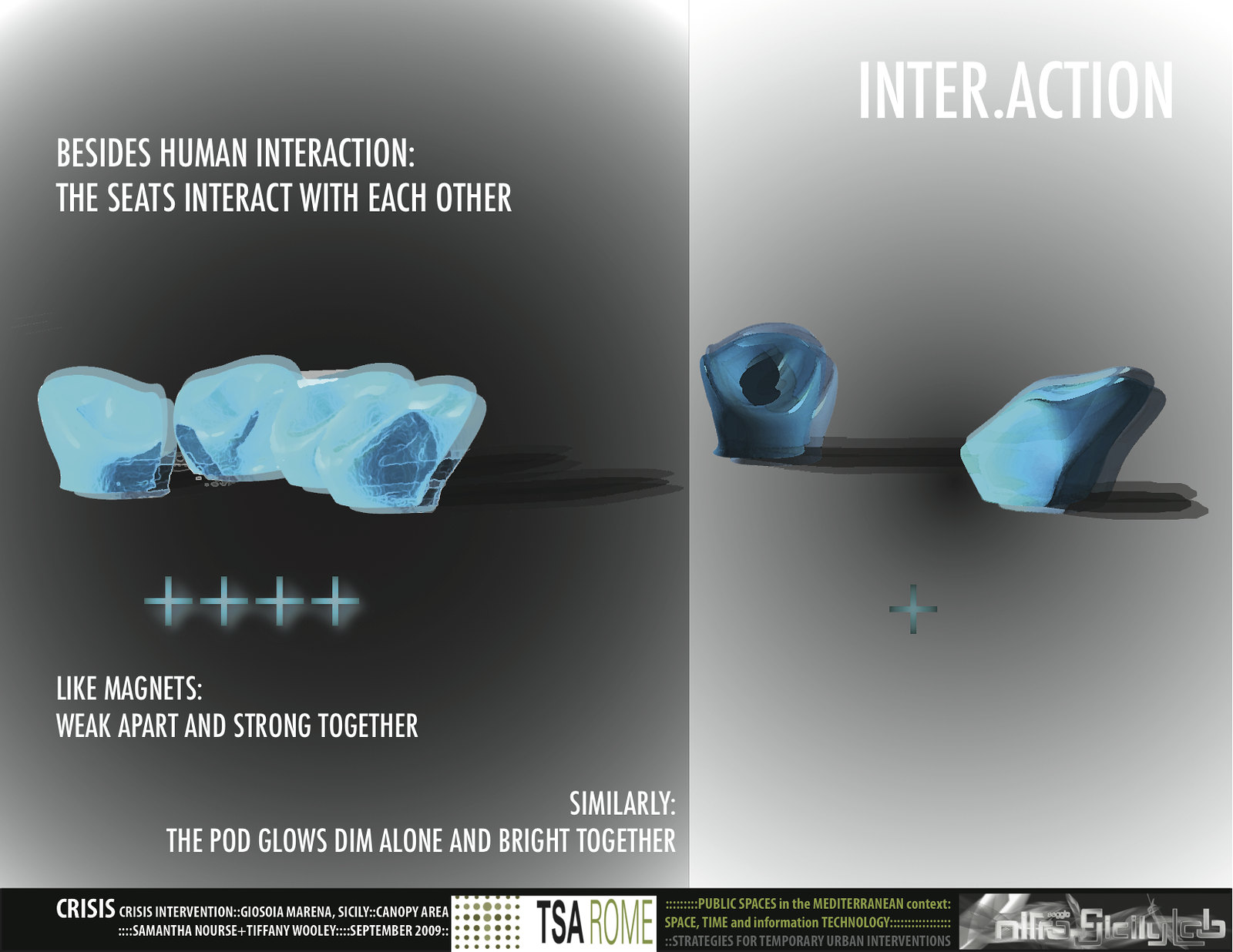The image is divided vertically into two halves. The left half has a dark gray background featuring white text at the top that reads, "Besides human interaction, the seats interact with each other." Beneath this text, an image of four blue seats is displayed, accompanied by four blue plus signs underneath them. Towards the bottom of the left half, additional white text states, "Like magnets, weak apart and strong together similarly," and, "The pod glows dim alone and bright together." The right half of the image has a lighter gray background and showcases two more blue seats. Above these seats, in the top left corner, the text reads, "Inter.action." At the very bottom, spanning the width of the image, a thin border contains text mentioning "Crisis intervention" and other information divided into two rows and four sections. There are small details like green text and a gray, black, and white logo in the bottom right, including mentions of names and dates, like "TSA Rome," "Geosa Morena," "Sicily Canopy Area," "Samantha Norse, plus Tiffany Woolley," and "September 2009." The entire composition suggests a focus on seats' interactivity and crisis intervention within public spaces or urban contexts.